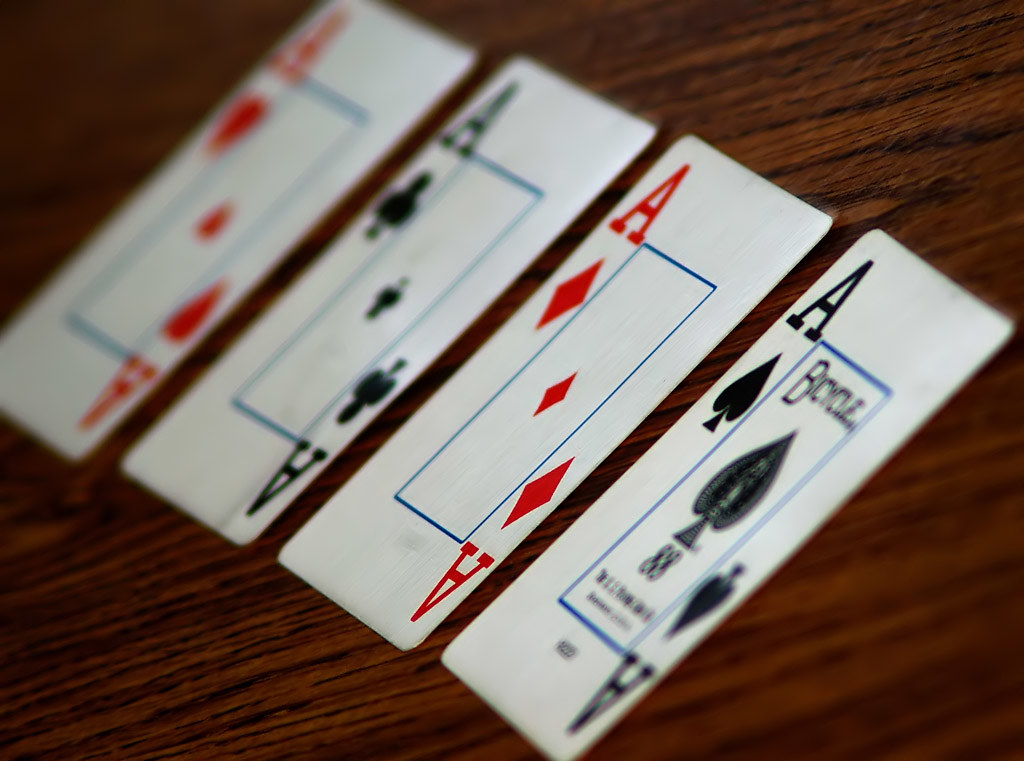Four playing cards lie spread out on a dark walnut wood table. These cards are all aces, arranged in a line from right to left. The sequence starts with the Ace of Spades, followed by the Ace of Diamonds, the Ace of Clubs, and ends with the Ace of Hearts. The cards become progressively blurrier as they move from right to left, with the Ace of Spades being the clearest. The first card prominently displays the "Bicycle" logo, indicating the brand. Despite some slight misalignments, the cards lay almost perfectly in line. The table is devoid of any other objects, emphasizing the focus on the four aces.